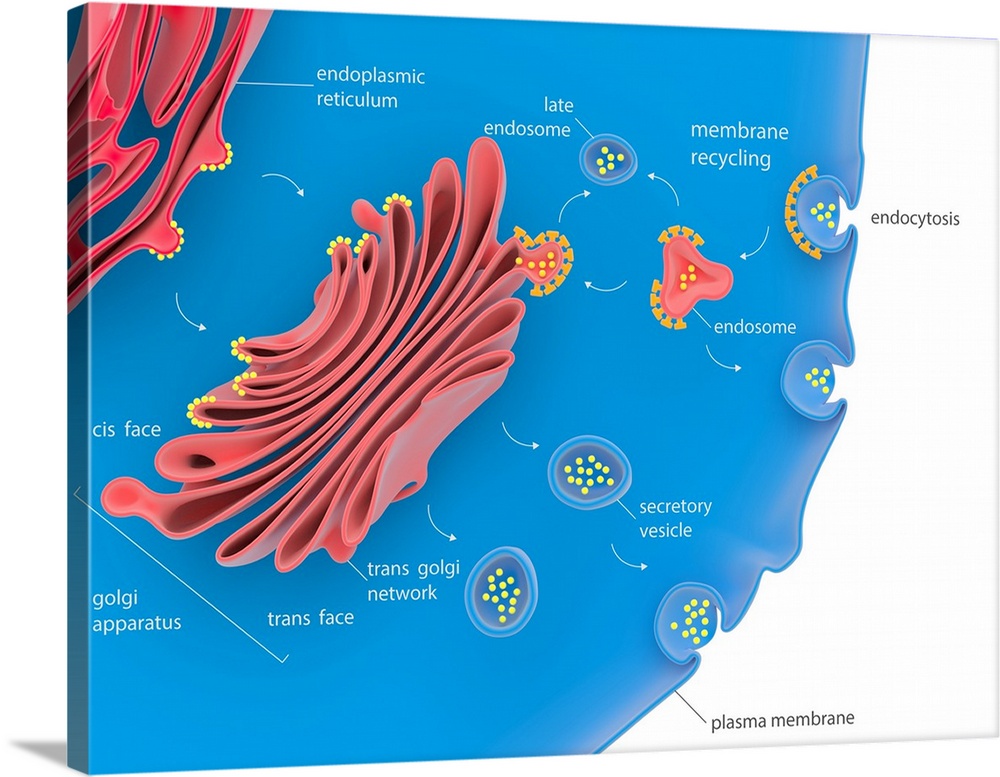This is a detailed educational illustration of a cell, depicted in a three-dimensional format as it wraps around the left-hand edge of the picture, giving it a volumetric appearance. Central to the image is a large blue cell, prominently featuring an array of intracellular components. 

On the left top corner, the endoplasmic reticulum is illustrated with a folded, layered structure akin to a croissant, colored pink against the blue background. Adjacent to this, the Golgi apparatus is displayed as a ribbony, red structure, highlighting the process of transfer from the Golgi to the plasma membrane. 

The illustration also includes various endosomes, with smaller yellow and red pieces labeled accordingly to indicate their roles in membrane recycling and endocytosis. Numerous vesicles and shapes punctuate the scene, such as secretory vesicles and the trans-Golgi network, each marked with indicative labels.

The right side of the image shifts to a lighter, possibly white area, where additional labels continue to delineate the detailed layout, reiterating the educational aspect of the illustration. This comprehensive diagram, likely sourced from a textbook on cell metabolism, offers a visually rich and labeled depiction of cellular components and their interactions.